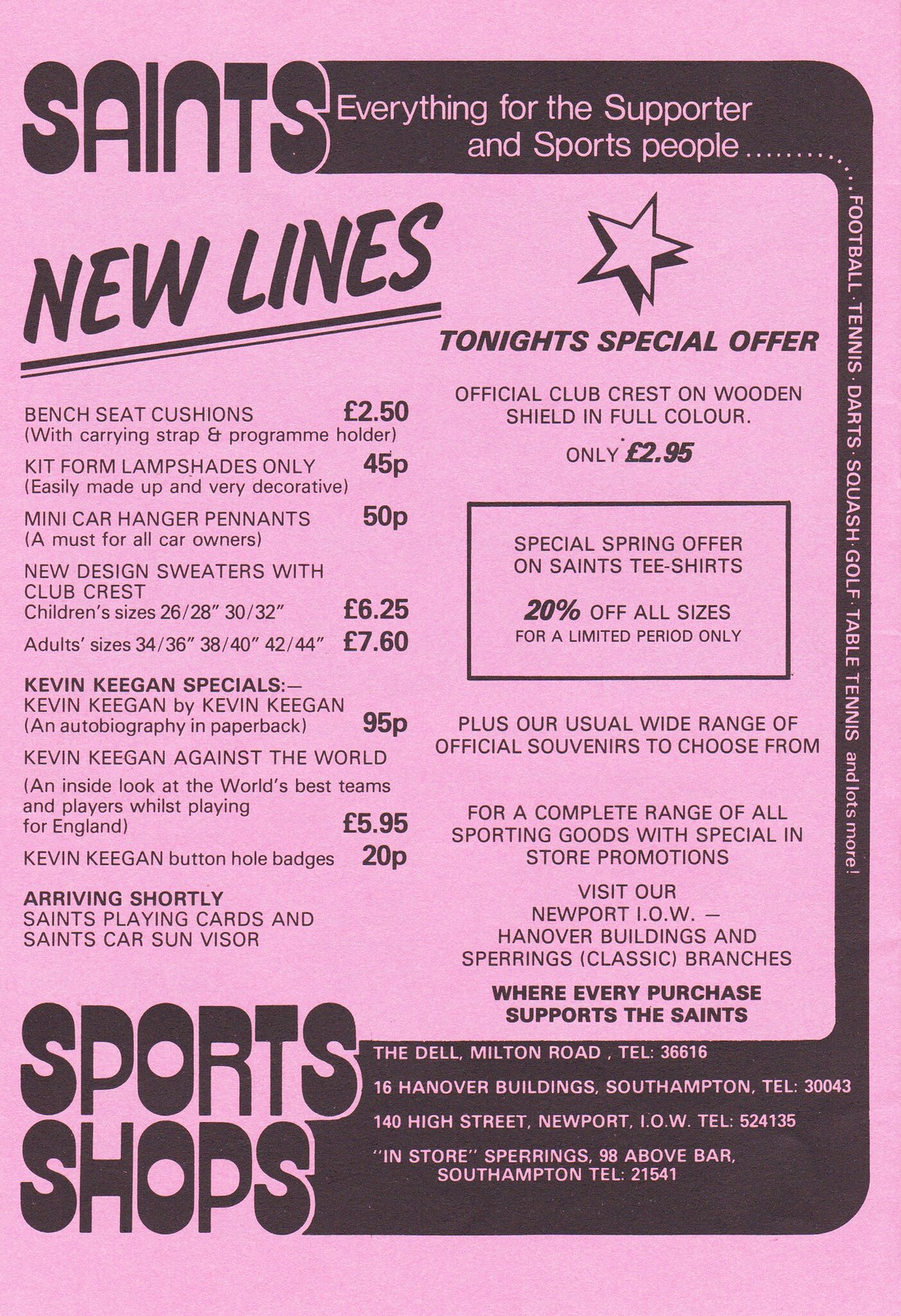The image is a vintage print advertisement printed in black ink on pink paper, featuring a variety of details relevant to sports enthusiasts. At the top, bold handwritten lettering reads "Saints" with an adjoining banner stating "Everything for the supporter and sports people." Along the right vertical edge, there is a list of sports such as football, tennis, darts, squash, golf, table tennis, and more.

The content is arranged in a portrait orientation with a comprehensive range of sports merchandise and specific items listed, such as new lines of bench seat cushions, kit form lampshades, mini car hanger pennants, and new design sweaters. A star outline highlights tonight's special offer, which includes official club crests on wooden shields in full color and a 20% off special on Saints t-shirts along with a variety of official souvenirs.

Across the bottom of the ad, contact information is provided for several store locations including the Dell, Milton Road, 16 Hanover Buildings, Southampton, 140 High Street, Newport, and Sparrings, located at 98 Above Bar, Southampton. On the bottom left corner, the words "sports shops" appear in the same typography as the title "Saints," emphasizing the range of available sporting goods and in-store promotions for sports supporters.